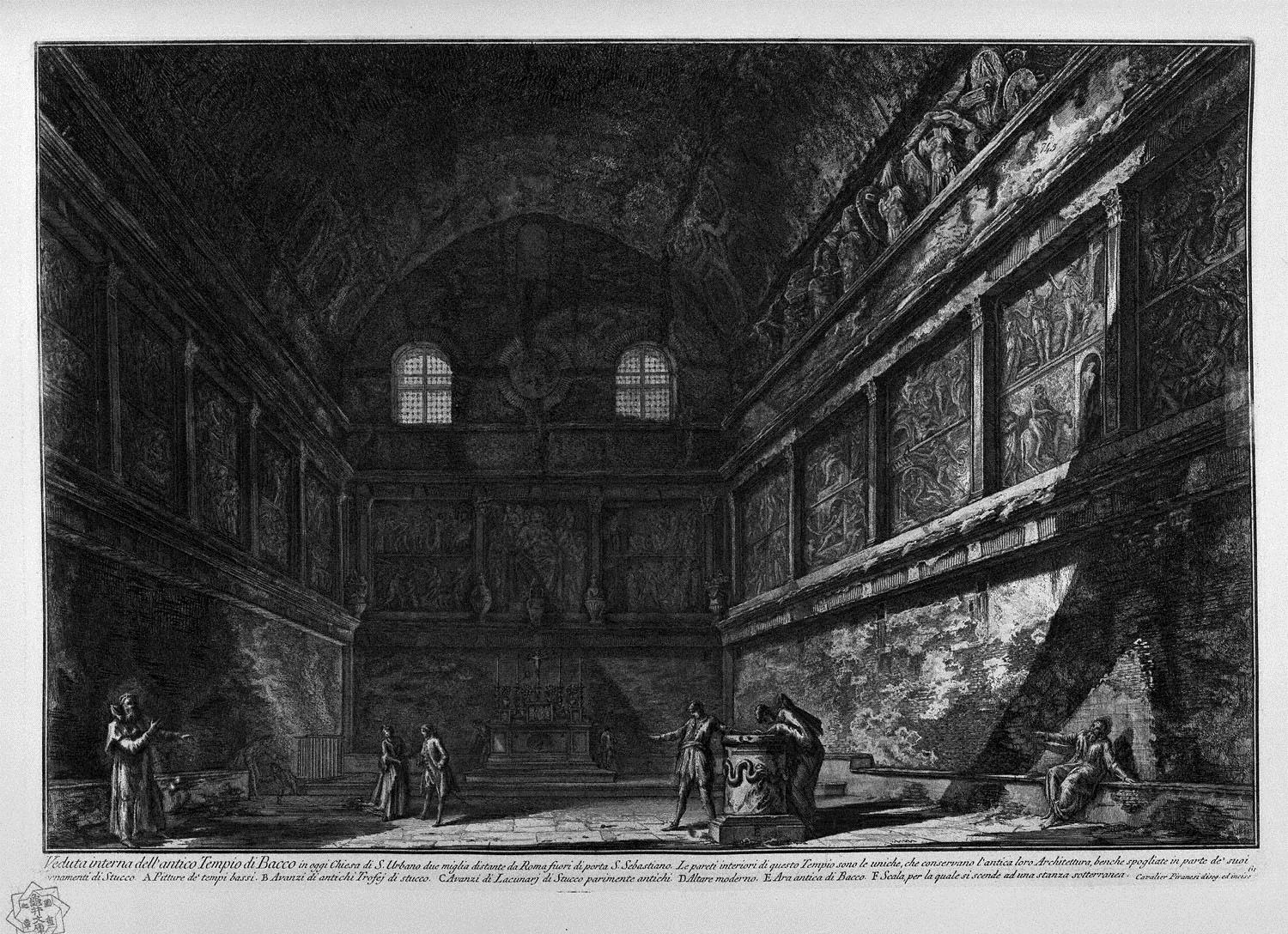The black and white image, reminiscent of a detailed charcoal drawing or sketch, portrays the interior of a grand, ancient structure, perhaps a 200-year-old house, castle, or temple. The immense room is adorned with intricate carvings along the walls, adding to its historical and artistic richness. In the background, two arched windows at the top center let in minimal light, emphasizing the shadowy ambiance. 

In the foreground, several figures populate the scene. On the right, a man, potentially wearing a long cape, bends over a fountain decorated with a snake motif, casting an ominous shadow on the wall behind him. Next to him, leaning against the wall, another figure, with skeletal features and open arms, suggests a haunting presence. To the left, a person who possibly appears to be a priest stands near the wall, while other indistinct figures, dressed in long gowns, gather centrally, adding to the room's eerie atmosphere. 

Along the bottom edge, ornate, unreadable text in another language adds a final touch of mystery to this elaborate and evocative scene.